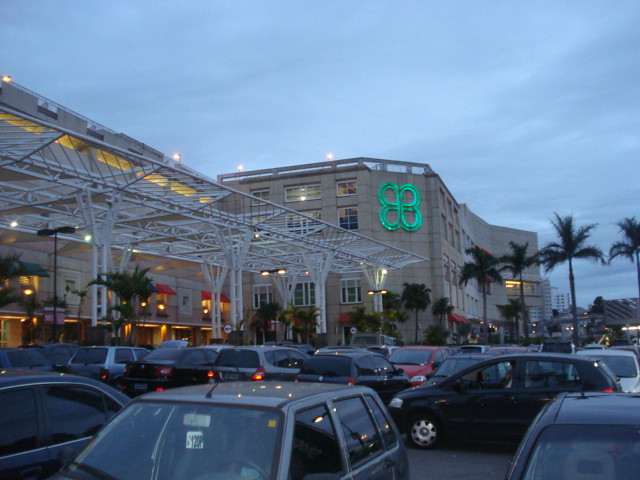In this early evening image, a large, light tan, four-story building with a white awning and a green, neon-lit clover-shaped logo stands prominently in the background. The building is well-lit with numerous lights, casting a warm glow as dusk approaches. In front of the building, an expansive parking lot is lined with palm trees and filled with numerous cars, some parked, while a few are in motion, including a dark blue car driving through and a black car searching for a spot. One car's red brake lights are visible, highlighting the twilight atmosphere under a somewhat cloudy sky. To the left side of the image, a patio area is observable, adding to the complex's inviting appearance.